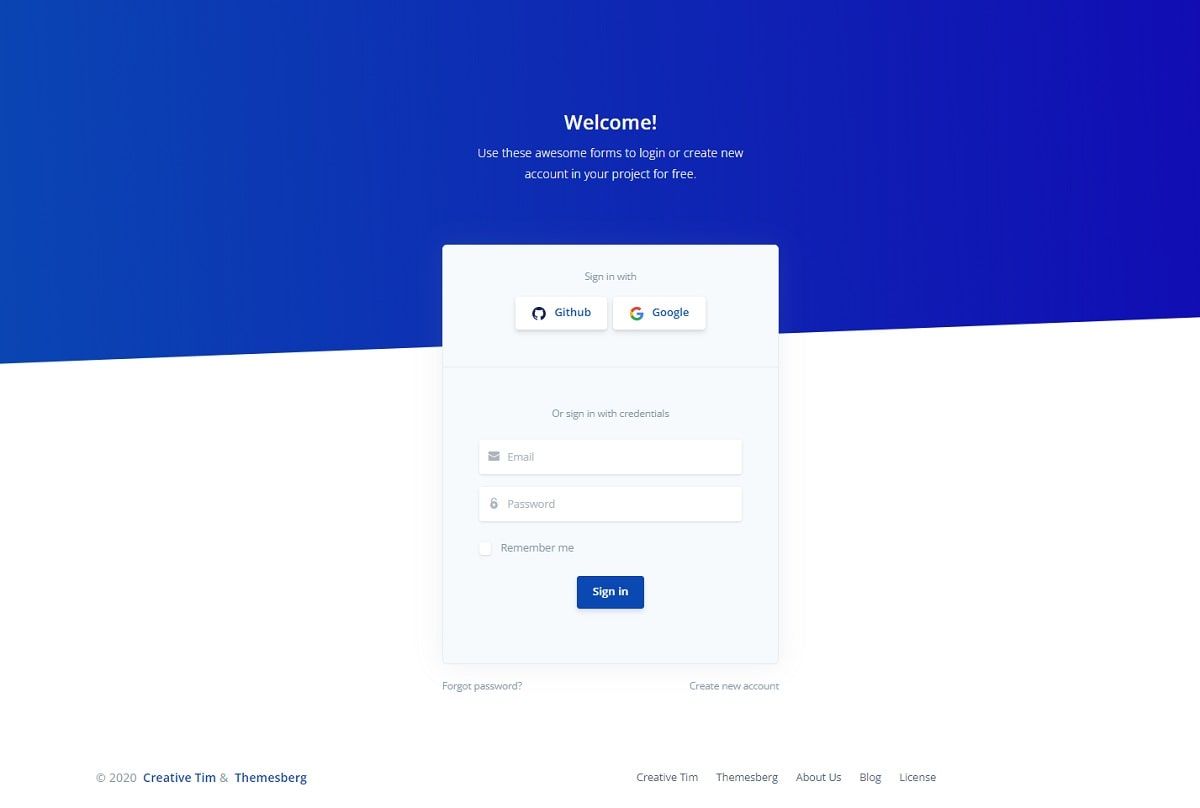**Screenshot Description: Detailed Login Page Overview**

The screenshot captures a login page divided into two distinct sections by a diagonal line. The top half features a blue background, while the bottom half is white. The diagonal line starts lower on the left side and ascends higher on the right side, creating a dynamic separation between the two colors.

Centered on the page is a white text box that straddles the blue and white backgrounds. At the top of this box, the text welcomes users with, "Welcome, use these awesome forms to log in or create your new account in your project for free." Below this welcome message, users are presented with two sign-in options, accompanied by their respective logos: "Sign in with GitHub" and "Sign in with Google."

Following these options, the login form offers a more traditional approach with the heading "Or sign in with credentials." Users can enter their email and password in the provided fields. There is an option to remember the login details via a "Remember Me" checkbox, which is not checked by default. At the bottom of the form, a "Sign In" button allows users to proceed with their login.

Underneath the white text box, there are two additional links: "Forgot password?" and "Create new account," giving users further navigational options.

Beyond the main login form, at the bottom-right corner of the page, there is a footer with copyright information reading, "© 2020 Creative Tim and Themesburg." To the right side of the page, a vertical menu offers further links: Creative Tim, Themesburg, About Us, Blog, and License.

Overall, the page design is clean and straightforward, focusing on simplicity and ease of use for logging into the application.